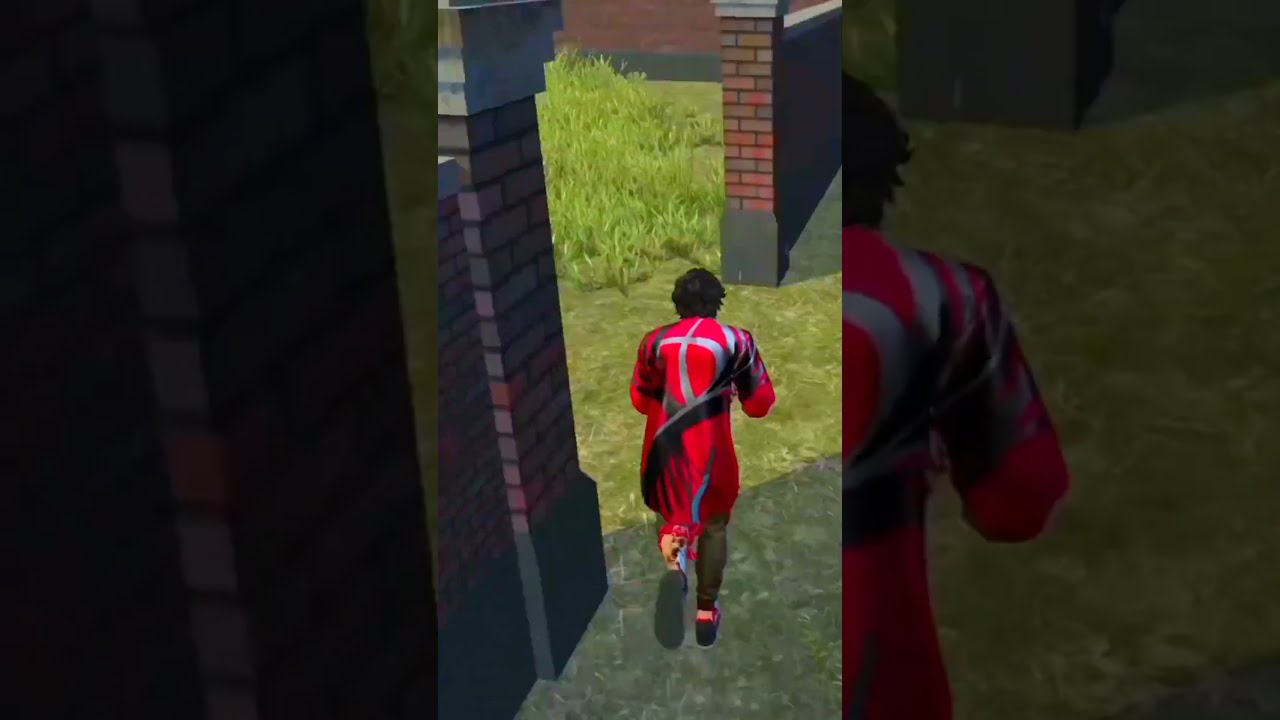The image is a detailed screenshot from a video game, featuring a young male character prominently displayed in the center. This central figure, dressed in a red and white outfit with grey pants and shoes, has his back towards the viewer as he runs towards a large, brick wall with an arched gateway. The character, who has black hair, appears to be in motion, with his running stance suggesting urgency or stealth. Surrounding the main image, the background is filled with darkened and zoomed-in versions of this central scene, creating a layered, immersive effect. Beyond the brick arch, lush green grass and bushes can be seen, hinting at an outdoor setting. The image conveys a moment of action or transition, with the character poised to move through the archway in an adventure or RPG game context.